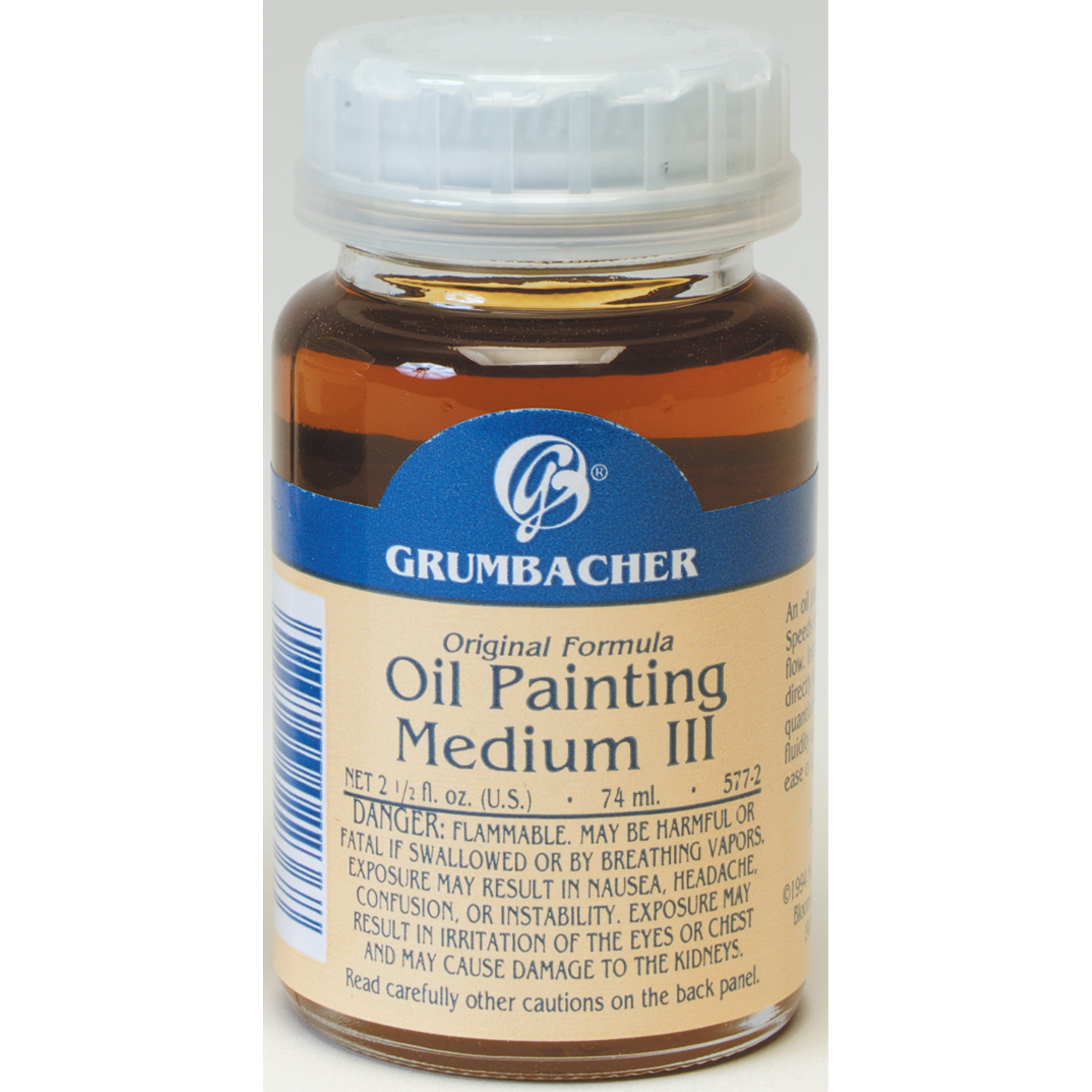The image features a photorealistic depiction of a 2.5 fluid ounce (74 mL) bottle of Grumbacher's original formula oil painting medium 3 against a light grey backdrop. The small bottle, approximately 4 inches in height, dominates the frame with its distinctive shape—an elongated sphere that is slightly flattened. It contains a transparent, thick, reddish-brown liquid. The bottle is sealed with a white safety cap, which also has an additional plastic cap on top. The label at the front of the bottle features the brand name "Grumbacher" at the top in blue, accompanied by their stylized "G" and "B" insignia. Below that, the text reads "Original Formula Oil Painting Medium 3" followed by warning messages including “Danger: Flammable,” and precautions about possible health risks such as nausea, headache, eye and chest irritation, and kidney damage. Additional information, barcodes, and other details are visible towards the right-hand curve of the bottle.